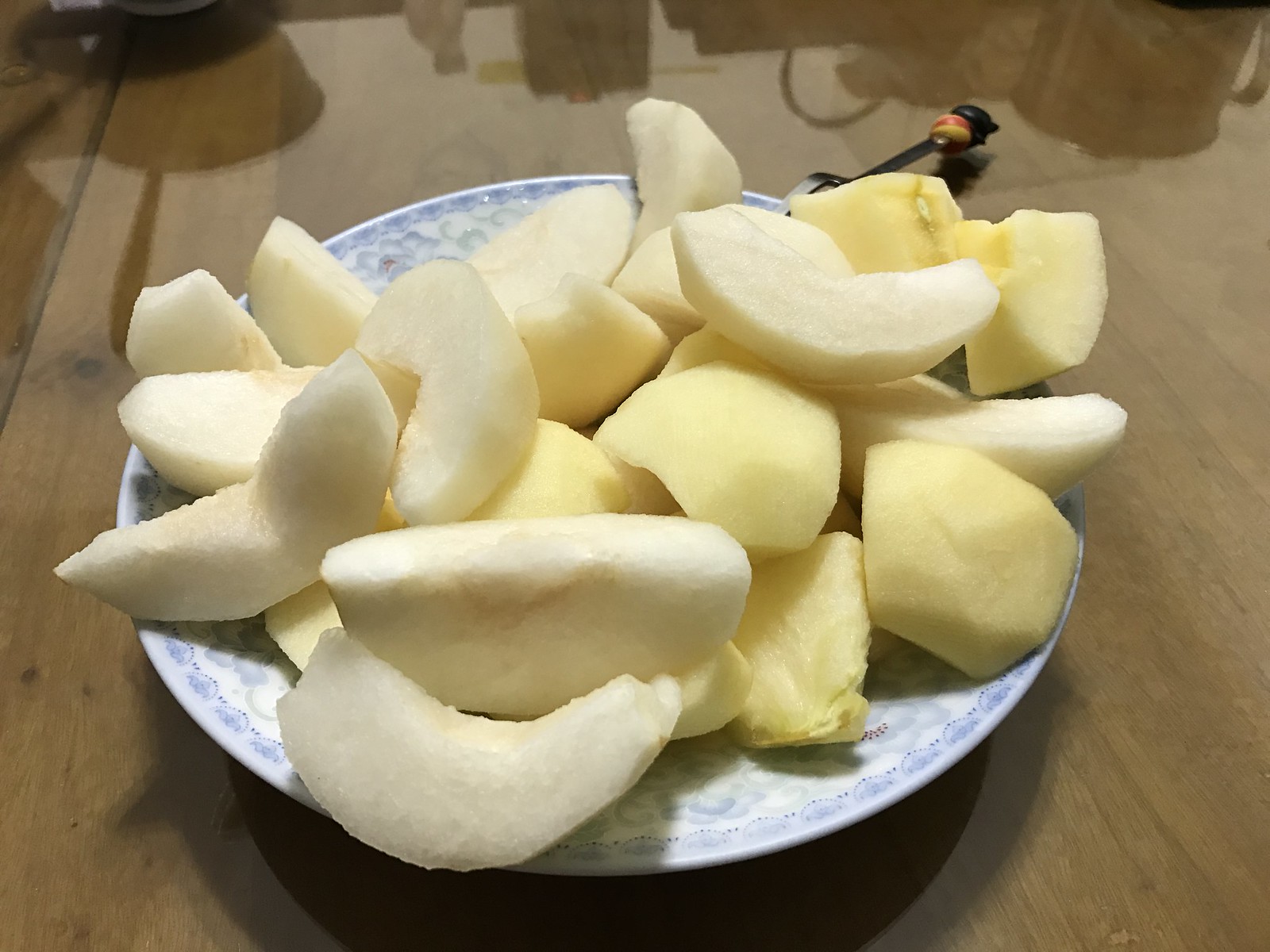This photograph captures a detailed view of a blue and white china plate, elaborately decorated with floral patterns, resting on a shiny, reflective medium wood table. The plate is heaped with an abundance of peeled and cored apple slices, varying in shades from pale white to light yellow, some with concave centers where the cores have been meticulously carved out. The sheer volume of fruit makes it look as if they might spill over the edges of the plate. At the right side of the plate, partially covered by the apples, lays a black fork with a wooden bead handle extending off the plate and onto the table. In the upper part of the image, the glossy table creates reflections of various shadows, hinting at other objects and appliances in the surrounding space.